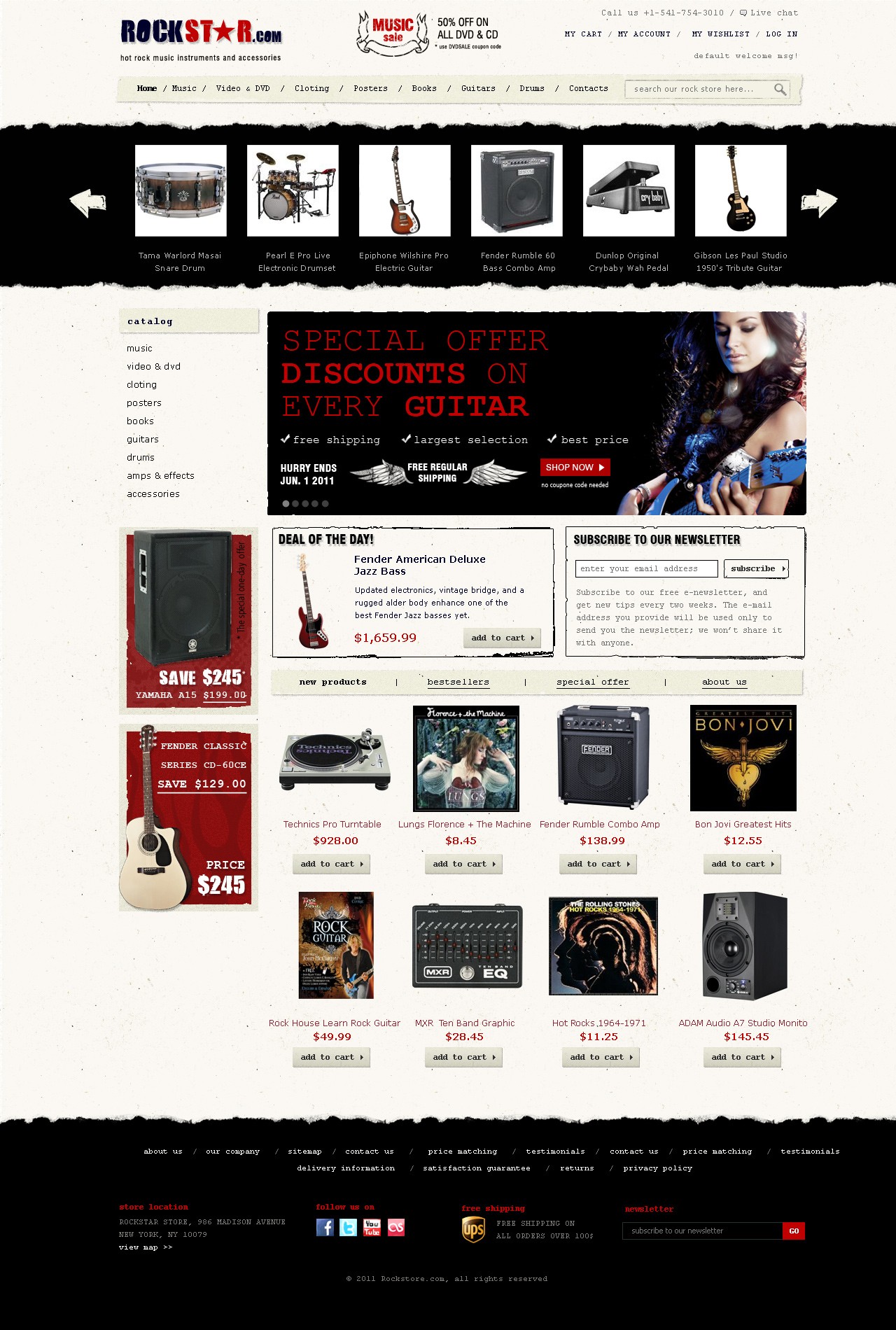The website rockstar.com is showcased with a prominent logo in the top-left corner. At the top center, a banner announces a significant sale: "50% off on all DVDs and CDs." Just below this banner, there is a tan navigation bar with various tabs, though the text is too small to decipher, along with a search bar.

A central feature of the website is a black box displaying different musical instruments depicted in white icons. Users can navigate through these instruments, which include a drum set, guitar, amplifier, pedal, and another guitar, using arrows on the left and right sides of the box.

Below this section, an image of a woman playing a guitar is accompanied by a caption that reads "Special Offer: Discounts on every guitar." Additional text, though too small to read, accompanies this offer. Adjacent to this is a box titled "Deal of the Day," highlighting an American Deluxe Jazz Bass. This section includes further text that is not legible, alongside an "Add to Cart" button.

Further down, there's an invitation to subscribe to the newsletter, with a box provided for email entry, followed by additional small text. On the left side of the page, a vertical column lists various categories such as "Catalog," "Music Video and DVD," and "Strings," though the text remains minuscule.

There are also prominent advertisements, including one for an amplifier with savings of $245 and another for an acoustic guitar listed at $245. The website displays various products in search results, including a turntable, CD, amplifier, book, mixer, another CD or vinyl, and a speaker.